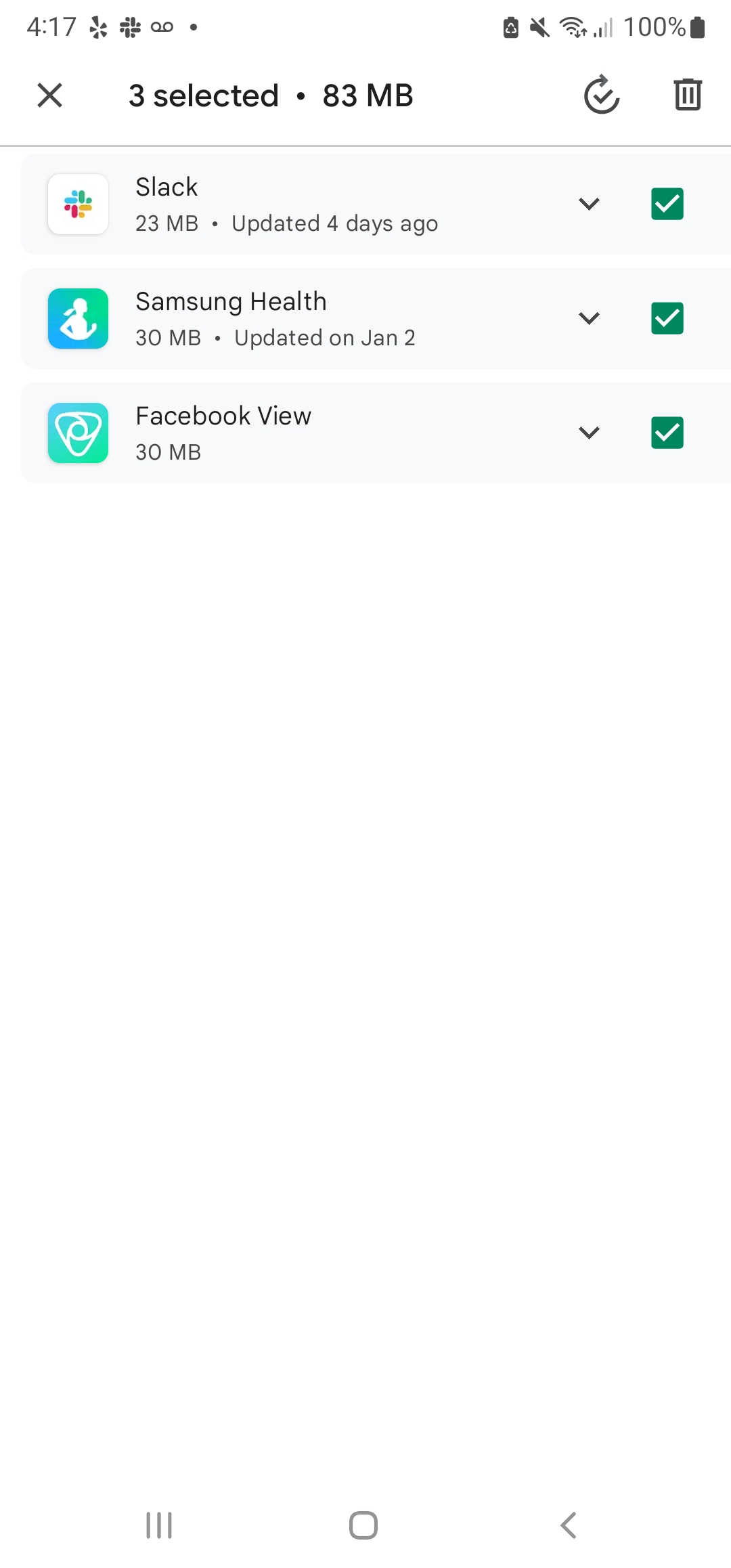Screenshot of a smartphone display featuring an interface in battery saver mode. The device is connected to Wi-Fi with two signal bars and has a 100% battery charge. The status bar shows no sound notifications are enabled.

The main screen shows a file management menu where three items are selected. The files are listed with detailed information: 

1. **Slack** - 23 MB, represented by a four-leaf clover icon with blue, green, red, and yellow colors.
2. **Samsung Health** - 30 MB, depicted with an icon showing a woman on a light blue background.
3. **Facebook View** - 30 MB, represented by an icon resembling a triangle with a design similar to the Google Chrome emblem in the middle.

Below these files, there are options to cancel the selection, refresh the list, or delete the selected items. The actions are confirmed by checkmarks next to each file, indicating they are ready for deletion.

At the bottom, the on-screen navigation buttons include (from left to right) the menu button, home button, and back button.